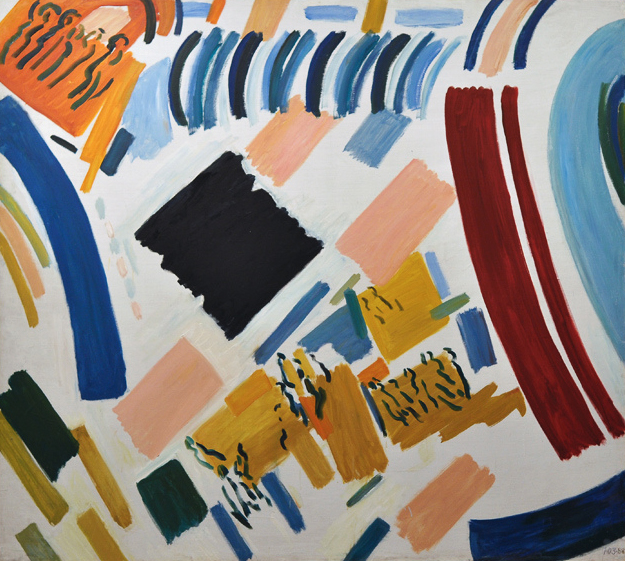The image is an abstract acrylic painting on a predominantly white background. It prominently features geometric shapes, primarily squares and rectangles, with an array of colors including black, tan, blue, green, red, orange, and pink. The shapes are arranged without a discernible pattern, some appearing as quickly drawn smudges or finger paintings. In the top left corner, there's an orange square, while the middle showcases a black square. To the right, a striking red streak or vertical curve separates the rectangular shapes from what seems to be more circular or arced forms, indicating this might be a smaller section of a larger composition. Additional blue curves are found in the bottom right and near the top left. The bottom right corner also bears the date "10382." The painting's overall aesthetic is dynamic and chaotic, with various dimensions and orientations of rectangular forms interspersed with arced shapes, lending it a vibrant, playful quality.